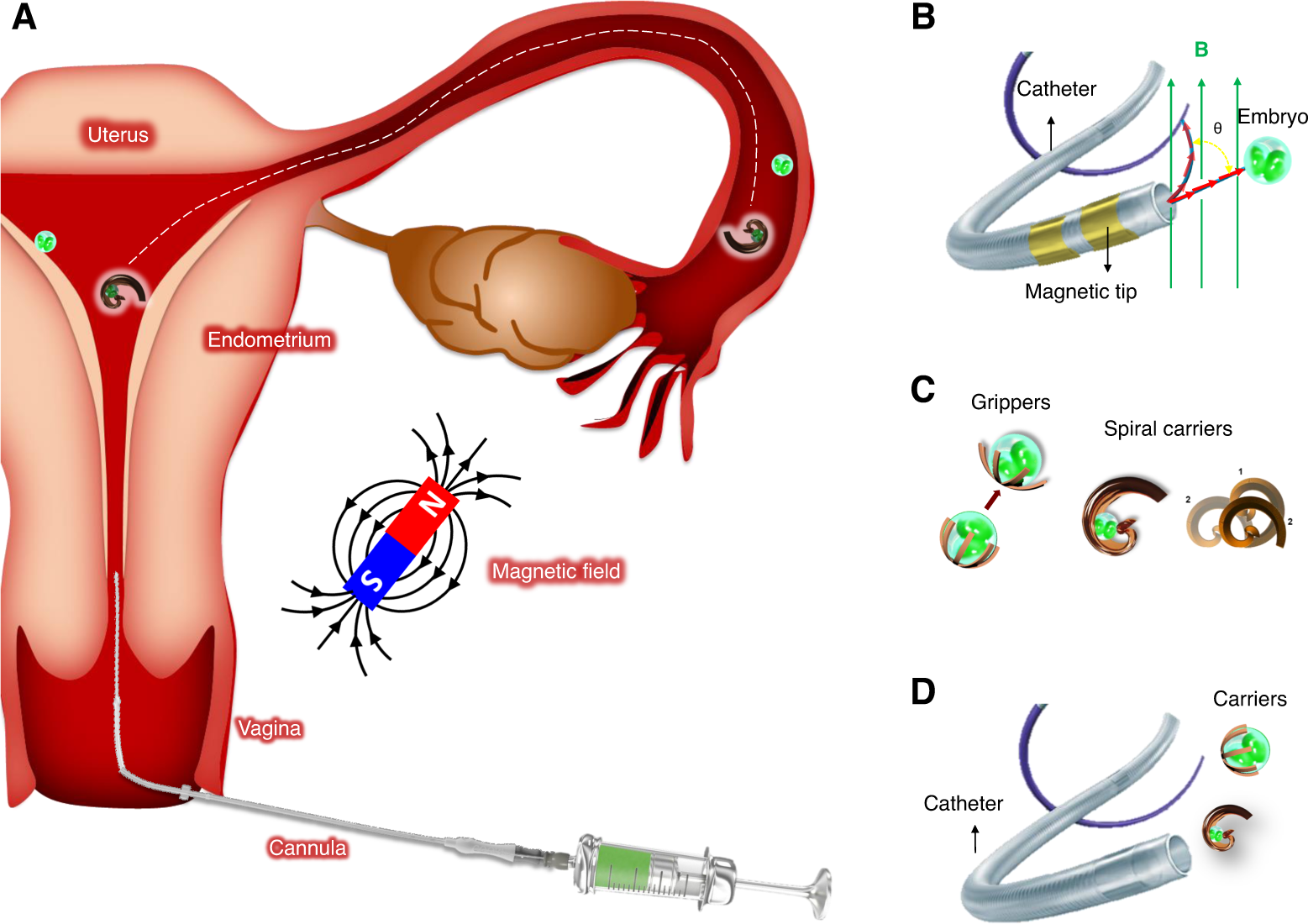The image is a detailed scientific diagram against a white background, illustrating aspects of female internal anatomy and various medical instruments. At the top left corner, labeled with the letter 'A', there is a diagram of a uterus depicted in shades of peach and red. The uterus is connected to fallopian tubes, and at the bottom, an intravenous-like tube is shown, possibly injecting an orange liquid. To the right of the uterus, there is a section labeled 'S' in blue and 'N' in red, indicating a magnetic field.

In the upper right corner, letter 'B' denotes an image of a catheter with a magnetic tip around an embryo. Below this, labeled 'C', are illustrations of grippers and spiral carriers. Finally, at the bottom right, letter 'D' showcases an image of catheter tubing and carriers. The diagram is likely explaining medical procedures involving uterine instrumentation and the use of catheters and magnetic tools.